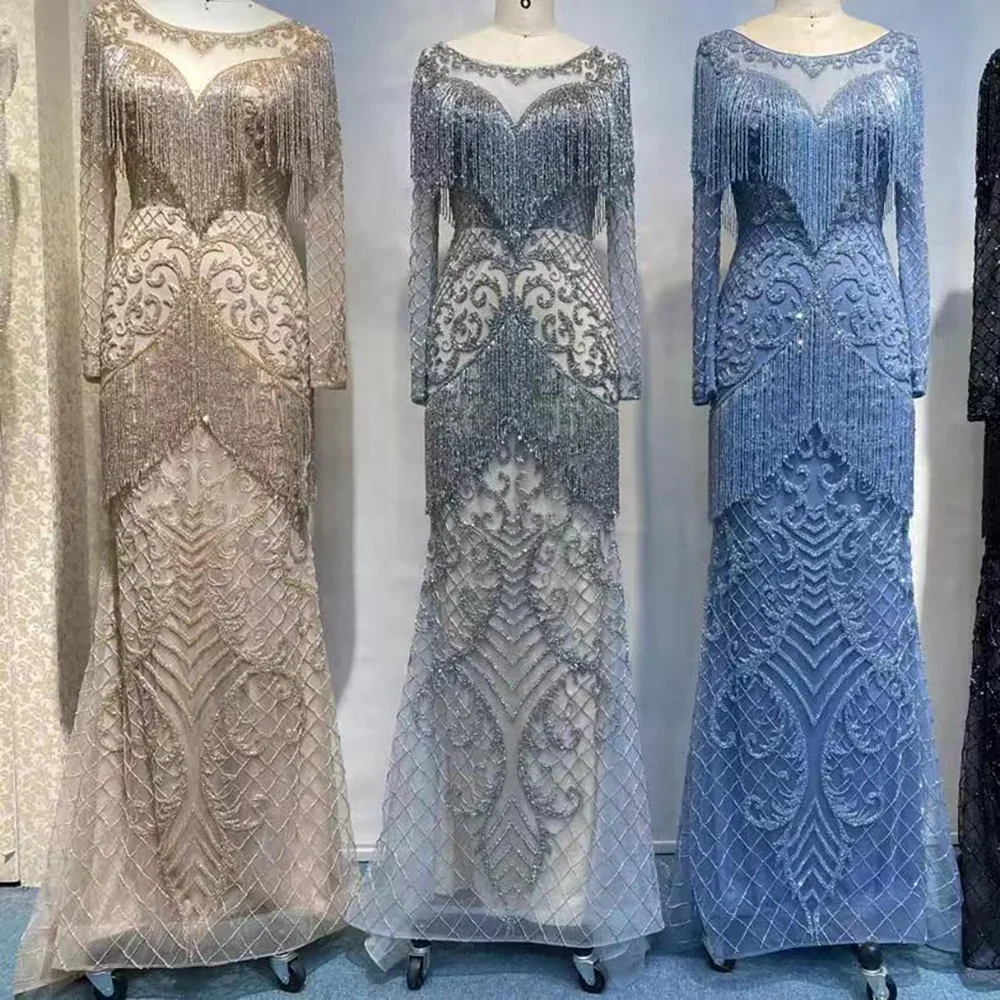This photograph showcases three elegant, long-sleeved dresses that, while identical in cut and design, differ in color. The dresses feature intricate swirl patterns and are adorned with hanging beads around the waist and chest area. Each dress, with its rounded neckline, stretches down to ankle length. They are displayed on a stark, hard white mannequin, covered in a shiny reflective plastic, that stands on four black rubber caster wheels with silver brackets, allowing for mobility. The mannequins are aligned against a white wall, set on a blue carpeted floor. The dress on the left is a light tan, the middle dress is a light gray with hints of blue, and the dress on the right is fully blue. The overall setting offers a clear but simple background, emphasizing the elaborate and formal nature of the attire.